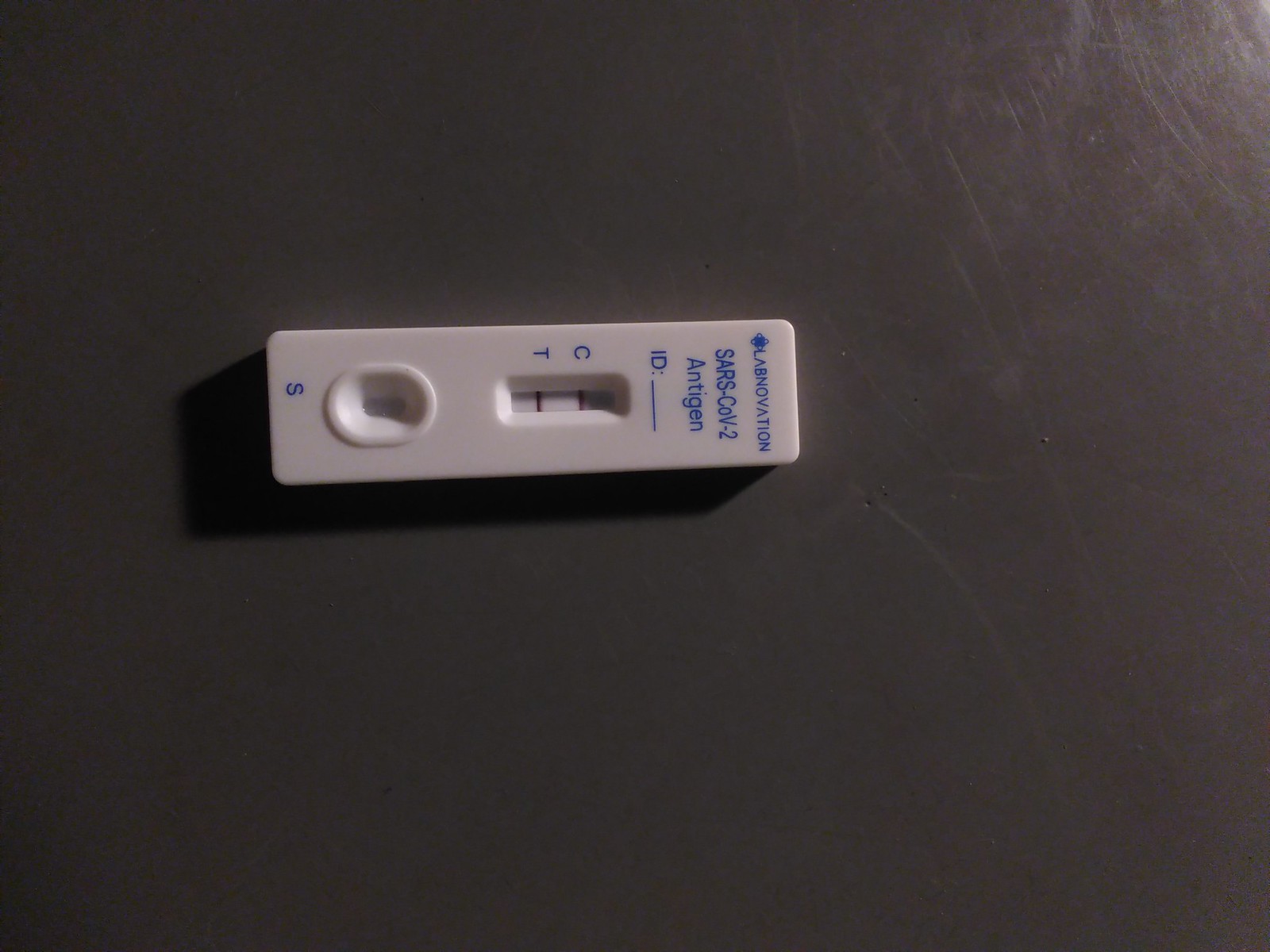An indoor, close-up, color photograph displaying a blood sampling test device placed on a black countertop. The device, rectangular in shape and approximately three inches long by one inch wide, is oriented with its bottom end to the left and top end to the right. The right side of the white plastic casing features the vertical text "Lab Novation." To the left, in capital letters, "SARS-COV-2" is prominently displayed, followed by the word "Antigen" below it. A label marked "ID:" with a blank line follows this text. 

Central to the device is a small rectangular window revealing two red lines. The line on the left is labeled "T," indicating the test line, and the line on the right is labeled "C," representing the control line. At the bottom end of the device, an oval slot intended for the blood sample is marked with an "S" below it. The test appears unused, as no visible blood sample is within the slot. 

A gentle light source from the upper right creates subtle shadows extending towards the left and lower left corners of the image. The overall composition indicates it is a diagnostic tool for detecting SARS-CoV-2 antigens. No other text or markings are visible.